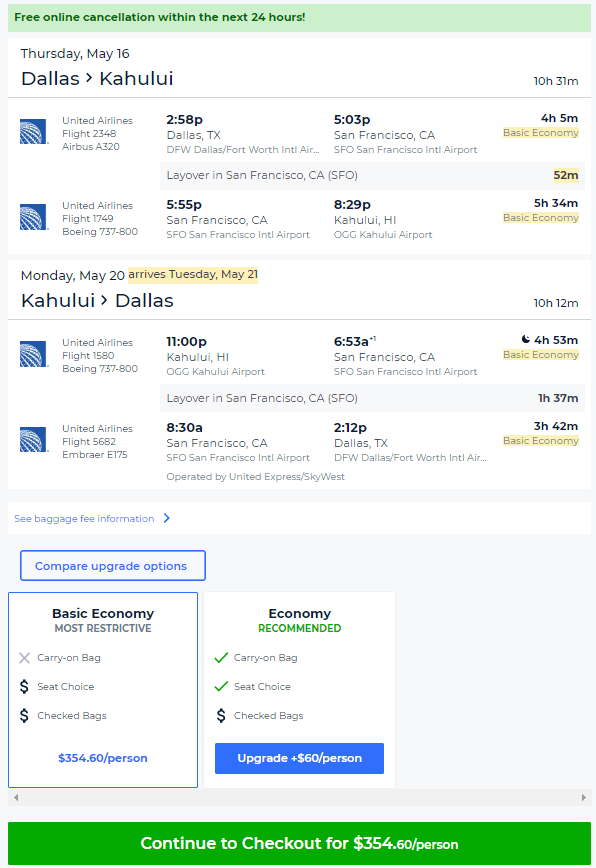The image displays a flight itinerary against a white background with black text. At the top, there's a prominent green box containing the message, "Free online cancellation within the next 24 hours." Below this, the itinerary details are provided. It specifies a flight on Thursday, May 16th, from Dallas to Kahului. The flight duration is listed as 10 hours and 31 minutes. The first leg is on United Airlines flight 2348, an Airbus A320, departing from Dallas Fort Worth International Airport (DFW) at 2:58 PM and arriving at San Francisco International Airport (SFO) at 5:03 PM. There is a layover of four hours and five minutes in San Francisco. The second leg of the journey is on United Airlines flight 1749, a Boeing 737-800. The end destination is Kahului, marked with a 52-minute basic economy layover.